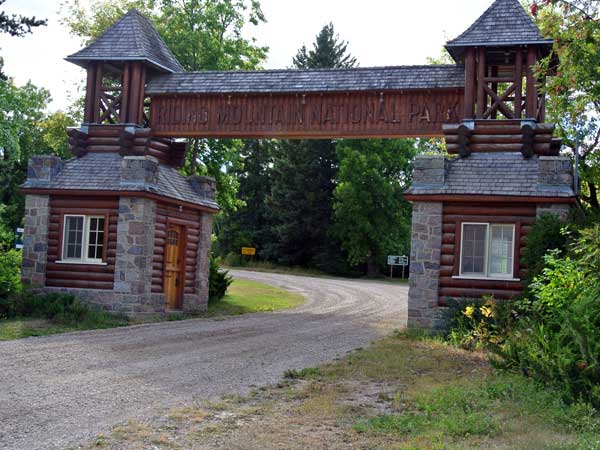This detailed photograph captures the entrance gate of Riding Mountain National Park. The entrance is flanked by two log cabin-style buildings on each side of a gravel road, connected by a large sign that reads "Riding Mountain National Park." The buildings are constructed with dark brown logs and light-colored stone bricks, each featuring windows and a distinct pointed roof. The road passes under the sign, coming from the bottom left of the image and curving to the left. The surrounding landscape showcases vibrant greenery, including bushes on the right and a background of trees, all illuminated by a sunny, summer day. Deep green grass and clusters of yellow flowers add to the picturesque scenery.